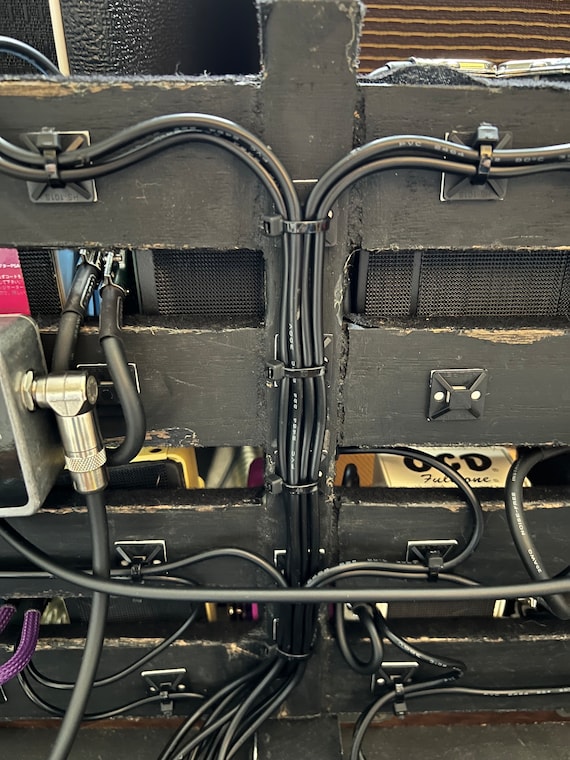The image depicts the back of what appears to be a vintage or abstract machinery setup, or possibly an art installation designed to mimic machinery. Central to the composition is a horizontally arranged wooden backboard with four distinct rows, each characterized by strategically placed gaps. These gaps reveal elements resembling the grill of a computer or a ventilation system. Attached to the wooden structure are numerous black wires, secured with plastic ties and metal or plastic bases, creating an intricate network that runs through the various sections.

The wires, numbering at least ten, converge from different directions: two from the left and two from the right in the topmost section, then meet and continue downward. This pattern repeats across the remaining sections. Notably, the third section also features a metal object connected to another black cord and a metal hose, enhancing the mechanical aesthetic.

Despite the detailed arrangement of wires, tubes, and vents, the setup doesn't appear functional and may serve a solely decorative or illustrative purpose. The image is highly detailed and photorealistic, capturing the texture of the wooden base, the shine of the metal components, and the tautness of the wires in striking clarity.